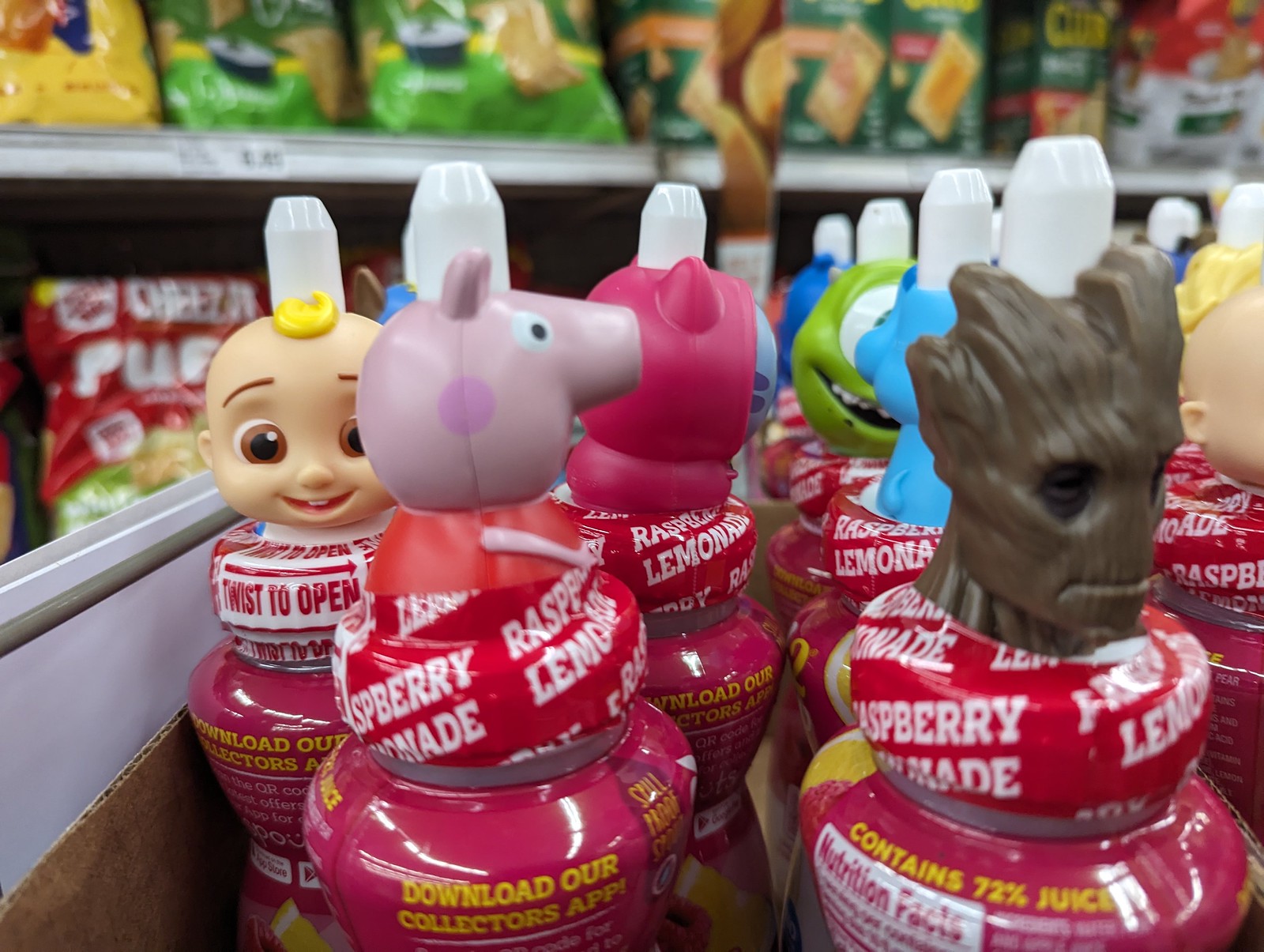The image captures a grocery store shelf stocked with an array of brightly colored, kid-friendly drinks. Each drink is encased in a plastic bottle adorned with various character heads as caps, ranging from animals to pop culture figures like Peppa Pig, Groot, and Hello Kitty. Most strikingly, all the bottles—with a visible count of around 10 or 11—seem to contain raspberry lemonade, indicated by consistent labeling and the mention of 72% juice content in yellow letters against a pink background. The caps come in diverse colors and designs, including a grotesque gray monster head resembling Frankenstein, a green figure with a weeping mouth, and a pig-shaped cap. Prominent words on the red background labels read "raspberry lemonade" and "twist to open." Panning out, the scene also includes a slightly out-of-focus background of grocery store shelves stocked with various bags of chips, including a distinguishable "Cheese It" bag. The main colors of the scene are pink, red, white, and green.